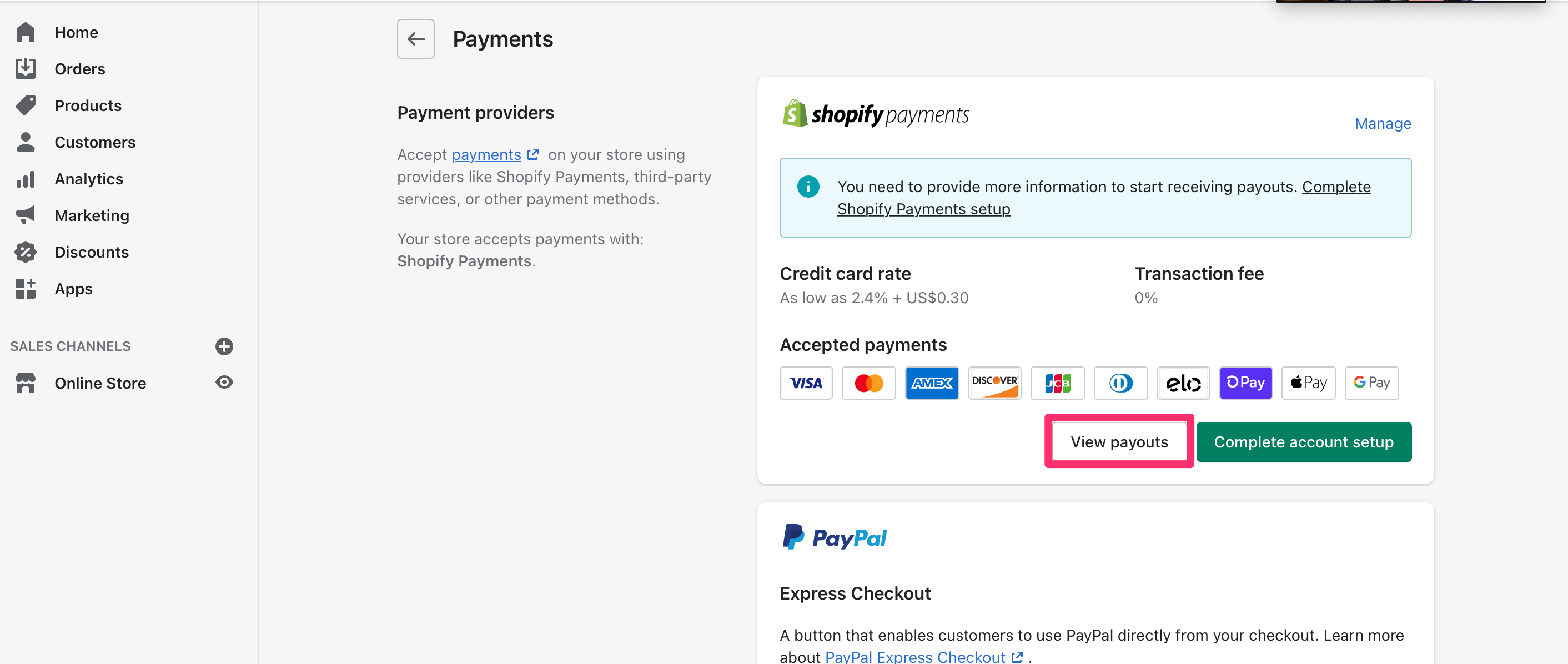**Descriptive Caption for Website Capture Image:**

The image is a detailed screenshot of a website interface, specifically focusing on the payment setup section of an online store dashboard.

On the left side, a gray sidebar menu features various navigational icons and labels, all in gray font. The menu items include:
- "Home" with a house icon
- "Orders" with a square icon
- "Products" with a price tag icon
- "Customers" with a person icon
- "Analytics" with bar icons
- "Marketing" with a bullhorn icon
- "Discounts" with a percentage icon
- "Apps" with square icons
- "Sales Channels" with a plus sign, "Online Store" accompanied by a storefront icon, and an eye icon

On the main section of the page, the header "Payments" is displayed in black font with a back arrow.

The subheading "Payment Providers" appears in gray, with the phrase "Accept Payments" featuring a clickable blue link to a detailed "Payments" page. An explanatory sentence follows: "Accept payments on your store using providers like Shopify Payments, third-party services, or other payment methods. Your store accepts payments with Shopify Payments."

Below this heading is a white square containing a green bag icon with a white dollar sign and the label "Shopify Payments." Accompanying this is a blue "Manage" link.

A blue notification box with a teal icon indicates: "You need to provide more information to start receiving payouts, complete Shopify payment setup."

Additional details listed include:
- "Credit card rate" as low as 2.4% + 30 cents per transaction
- "Transaction fee: $0.00"
- Accepted payment methods: Visa (blue), MasterCard (orange and red), Amex (blue and white), Discover (black and orange), and a series of colorful icons representing various digital payment methods like Apple Pay and Google Pay.

A pink-bordered box prompts users to "View Payouts," while a teal box urges "Complete Account Setup."

Finally, the page mentions "PayPal" in blue font, highlighting its logo, with a section about "Express Checkout" in black, explaining that this feature allows customers to pay directly via PayPal from the checkout page. A "Learn more" link provides further details about PayPal Express Checkout.